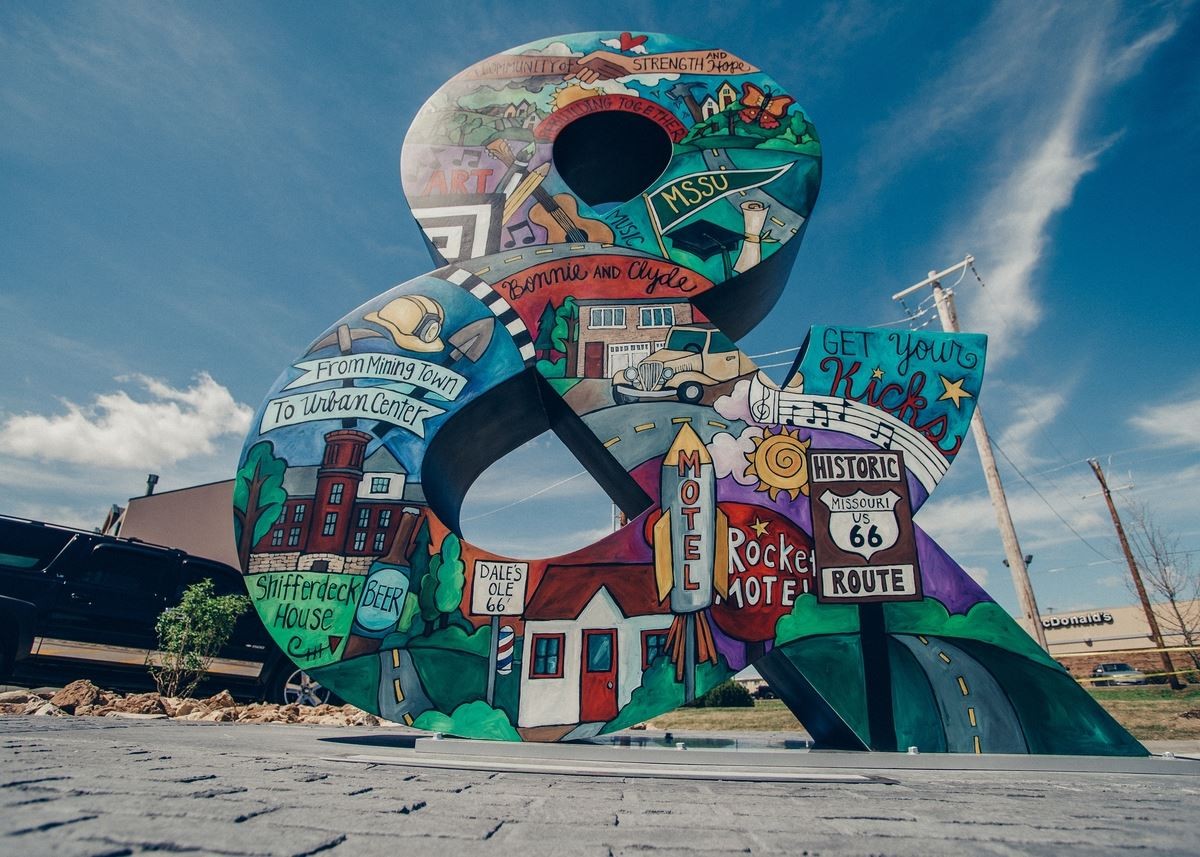This outdoor photograph depicts a large, three-dimensional sculpture in the shape of an ampersand (&), prominently situated on the ground and likely serving as a tourist attraction and historical marker. The surface of the ampersand is richly adorned with colorful paintings and illustrations that depict various elements and themes related to the area, possibly Missouri. Notable features include a house, road, rocket, sun, guitar, mining instruments, a butterfly, a hammer, and text such as "historic route," "get your kicks," and "Route 66." Specific references to local and historical points of interest are illustrated, including banners with "MSSU," "Community and Strength and Hope," "Bonnie and Clyde," "Mining Town to Urban Center," "Schifferdeck House," "Dale's Old 66," "Historic Missouri U.S. 66 Route," and a rocket labeled "Motel." In the background, several buildings are visible along with a McDonald's and a small shack, all under a clear blue sky with scattered white clouds.